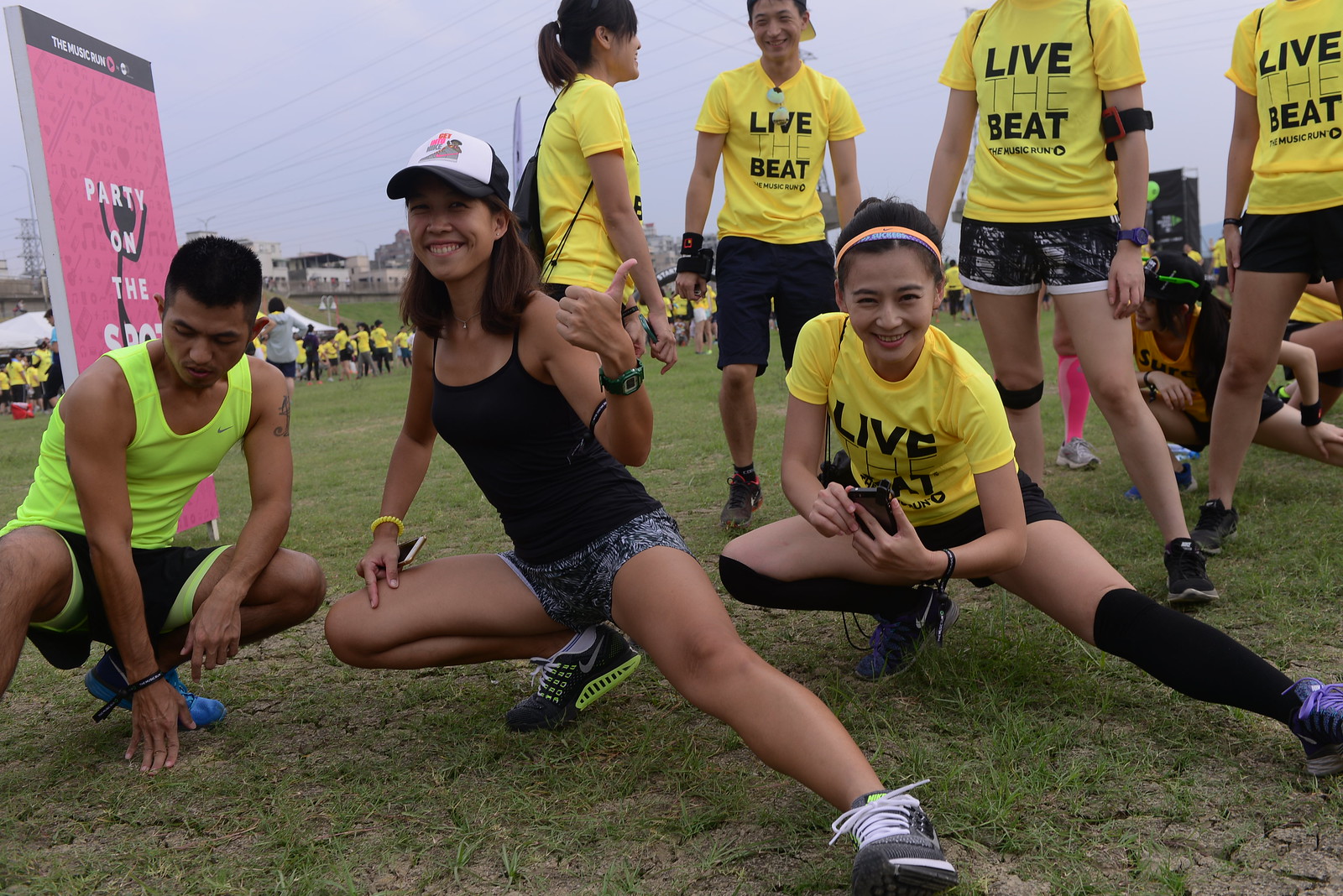The photograph captures a vibrant outdoor sporting event set in a hilly, open grassy field under a partly cloudy sky. At the forefront are seven young people, predominantly teenagers, involved in some sort of fitness activity or run. Three of them are squatting: on the left, a young man in a bright neon green vest stretches with his arm on the ground and looks down; in the center, a smiling young woman in a black tank top and black and white baseball cap gives a thumbs-up while holding her phone and squatting with one leg extended; on the right, another woman in the event's signature yellow "Live the Beat" t-shirt also squats, mimicking a stretch. Behind them stand four more individuals—both men and women—also clad in the yellow event t-shirts that read "Live the Beat, The Music Run." One girl, distinguishable by her pink bandana, beams directly at the camera. The field is teeming with other participants in matching yellow t-shirts, indicating a large turnout for the event. In the upper left corner of the image, a pink sign with white text declares "Party on the Spot," adding to the festive nature of the scene. The overall color palette of the image includes light blue, white, green, yellow, black, and pink, reflecting a lively and engaging atmosphere.